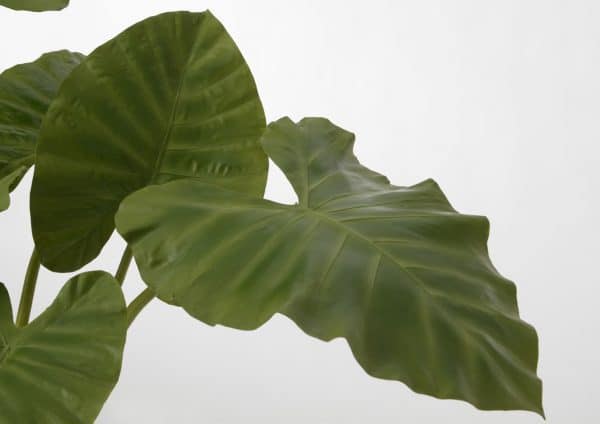The photograph captures a striking close-up of a green plant with large, heart-shaped leaves splaying out from the bottom left-hand corner, set against a minimalist white backdrop. The image, measuring seven inches across by five inches tall, features no additional text or borders, giving full attention to the plant's texture and form. The leaves exhibit a vivid green color with pronounced veins and a slight crinkle or wrinkled texture. The largest leaf, occupying a significant portion of the right side of the photo, is shaped like a spade, with pointed and V-shaped edges. Another leaf extends partially from the bottom left corner, pointing towards the corner, while additional leaves peek from behind, pointing upwards and to the left. Light reflects off the surface of the leaves, adding a touch of vibrancy to the otherwise simplified and lower-quality photography.